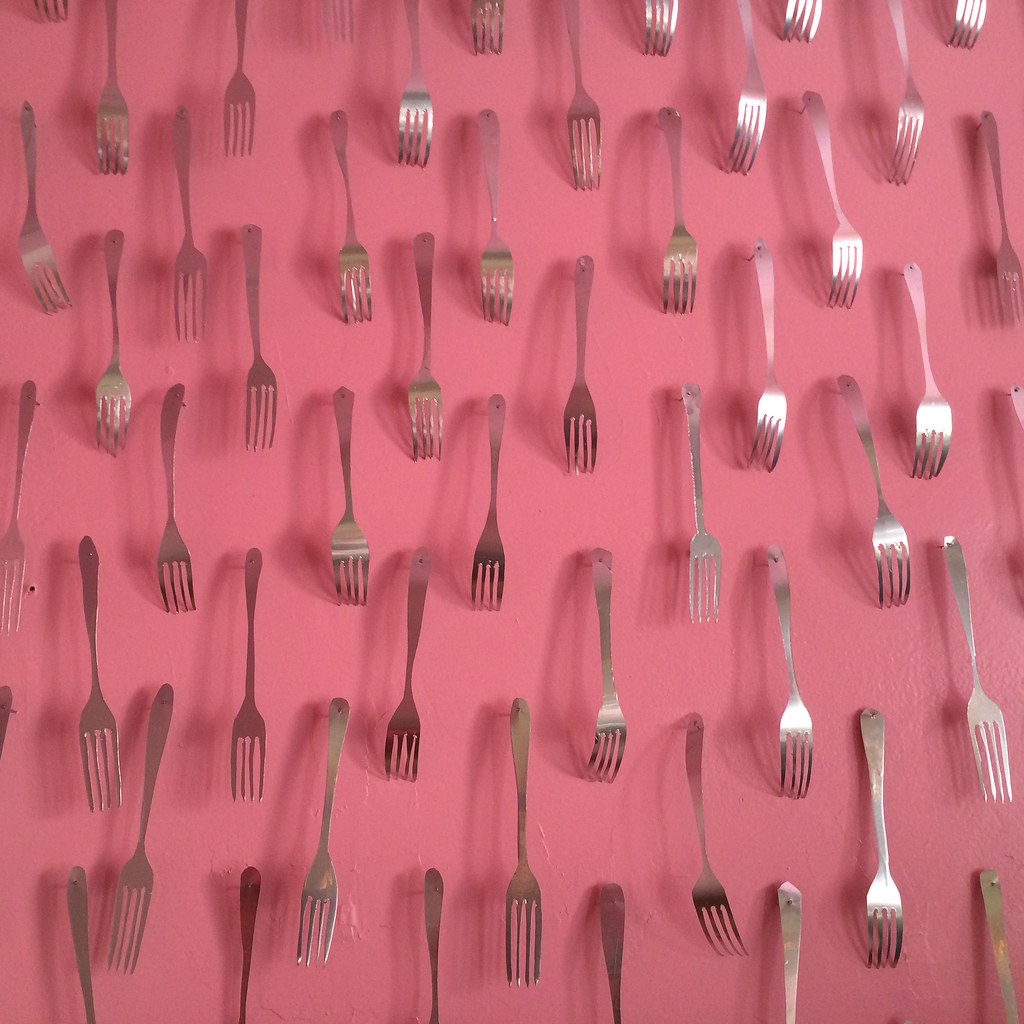This detailed photograph features an array of approximately 40 standard sterling silver forks placed haphazardly on a smooth, bubblegum pink surface, likely a table or tablecloth. The forks, casting prominent shadows, create a staggered diamond pattern, some positioned face down with the tines downward while others face up. Although they appear similar at first glance, a closer look reveals slight variations in the handles—some are rounded, some squared or diamond-shaped, and a few are more ornate. The forks are evenly spaced with decent gaps between them but not aligned perfectly, adding to the visually intriguing and somewhat chaotic arrangement. The right-hand side of the image shows the forks bathed in more light, highlighting their silver sheen and casting a glow that contrasts with the relatively darker, shadowed left side.